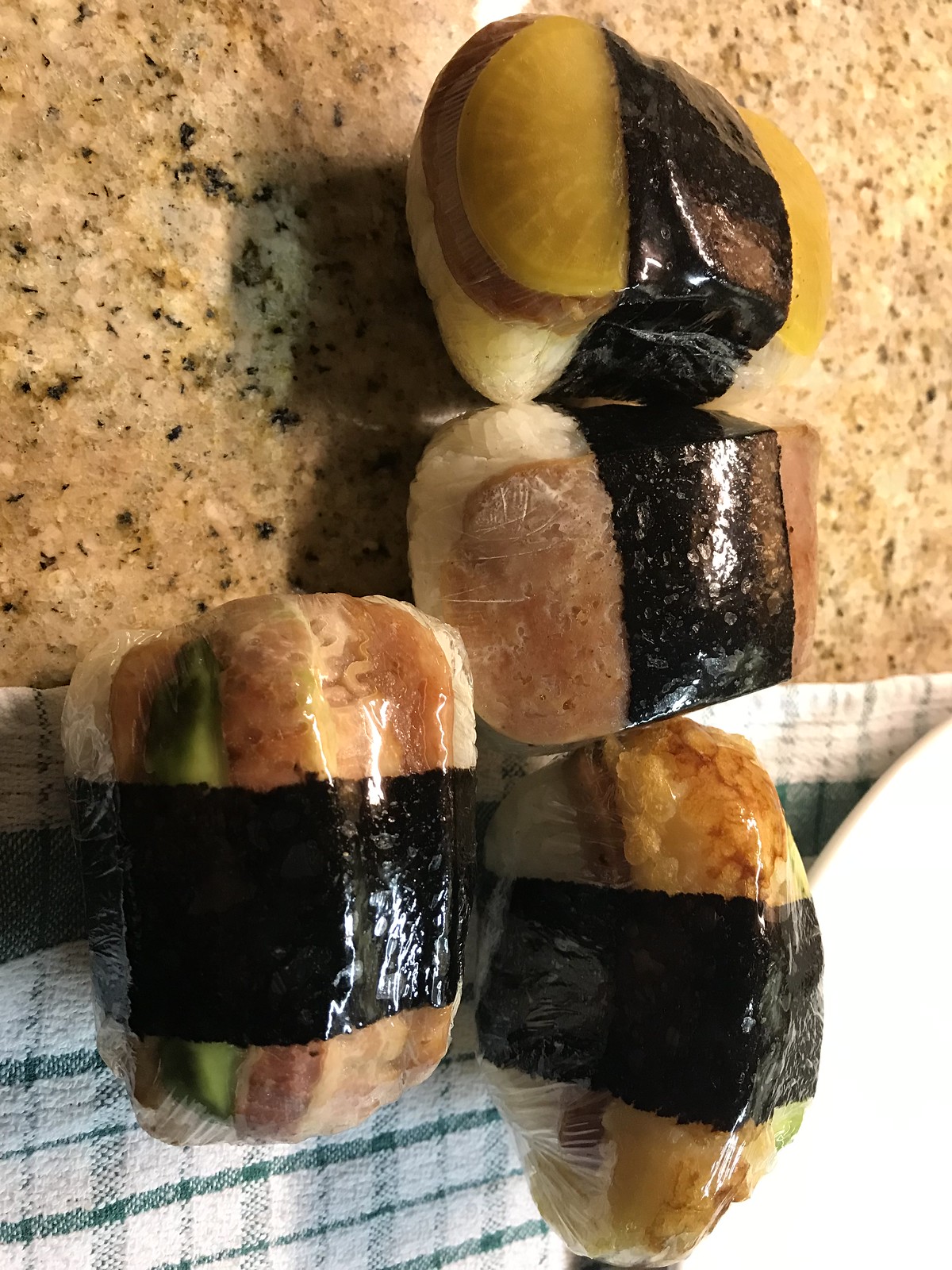This photograph showcases four large pieces of sushi set on a brown marble countertop with lighter brown and black speckles, partially covered by a green plaid-patterned towel. The image appears rotated 90 degrees clockwise. The sushi, wrapped in transparent plastic wrap, are placed next to a white plate in the lower right corner. Each piece of sushi features a vertical seaweed wrap, visible white rice, and an array of toppings. The top-left (originally upper) sushi includes light green pickle-like topping with brown meat underneath. The next piece, similar but without the green topping, also has a meat and rice combination. The lower left piece has brown meat, a vibrant green cucumber slice, and rice, while the lower right sushi piece showcases deep-fried dark and light brown elements, green in the back, and brown topping over rice.